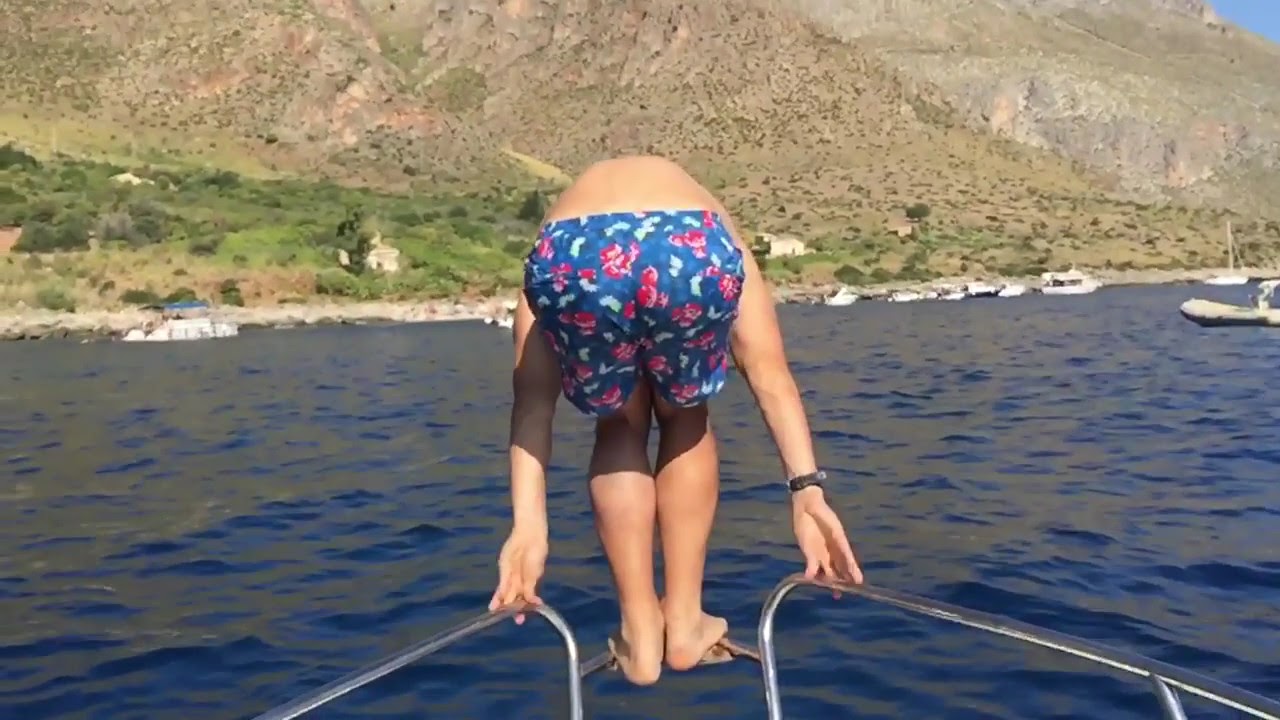The image depicts a young man, possibly a boy, standing at the front of a boat, poised to dive into the water. He is wearing blue swim trunks adorned with red flowers and green leaves. The scene captures him leaning forward, his hands gripping silver chrome bars that frame the boat's edge, and his feet firmly planted on a rounded metal pole connected to side bars, suggesting he is ready to leap. The deep blue water beneath him contrasts with the surrounding landscape, which includes lush green hills to the left and tan, rocky elevations to the right, encroaching from the shoreline upwards. In the top right of the image, a portion of the sky is visible. Other boats are scattered across the water, especially concentrated near the right shoreline. The background's mountainous terrain displays a mix of greenery and rocky gray surfaces, contributing to the scenic and adventurous atmosphere.